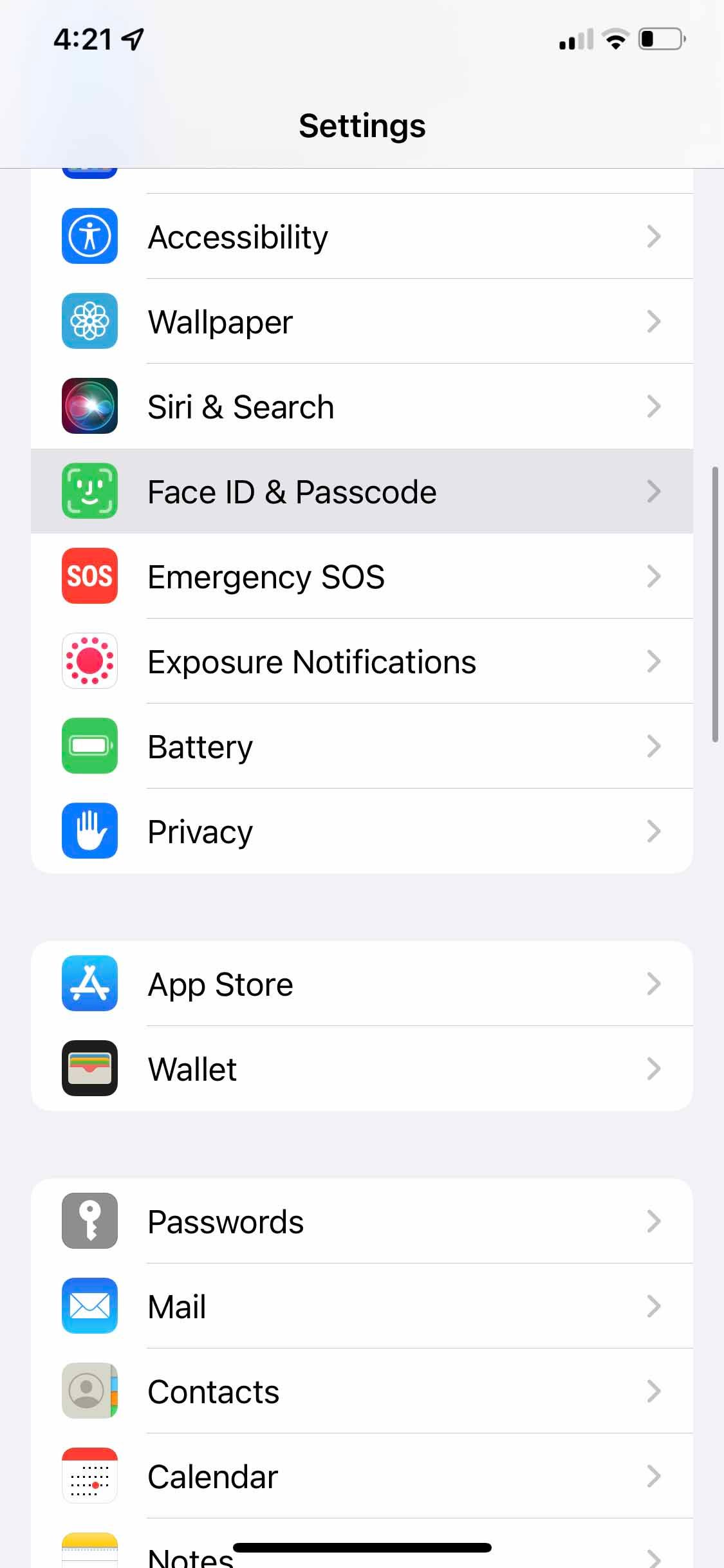This is a detailed screenshot of the settings menu on an Apple iPhone taken at 4:21 (AM or PM is not specified). The top bar of the screen shows standard icons: internet connection, signal bars, and battery level. The settings menu items are arranged vertically in the following order: Accessibility, Wallpaper, Siri & Search, Face ID & Passcode, Emergency SOS, Notifications, Battery, Privacy, App Store, Wallet, Passwords, Mail, Contacts, Calendar, and Notes. Each setting option is represented with an accompanying icon to its left and an arrow on its right, suggesting they are clickable to expand further. The menu is displayed with black primary text on a white background, except for the 'Face ID & Passcode' option, which is highlighted in gray. This gives the impression that it might be actively selected or in focus. Notably, there are light gray blank rows between 'Privacy' and 'App Store' and between 'Wallet' and 'Passwords', creating slight separations within the list. The icons are depicted in mostly primary colors, adding a visual distinction to each menu item.